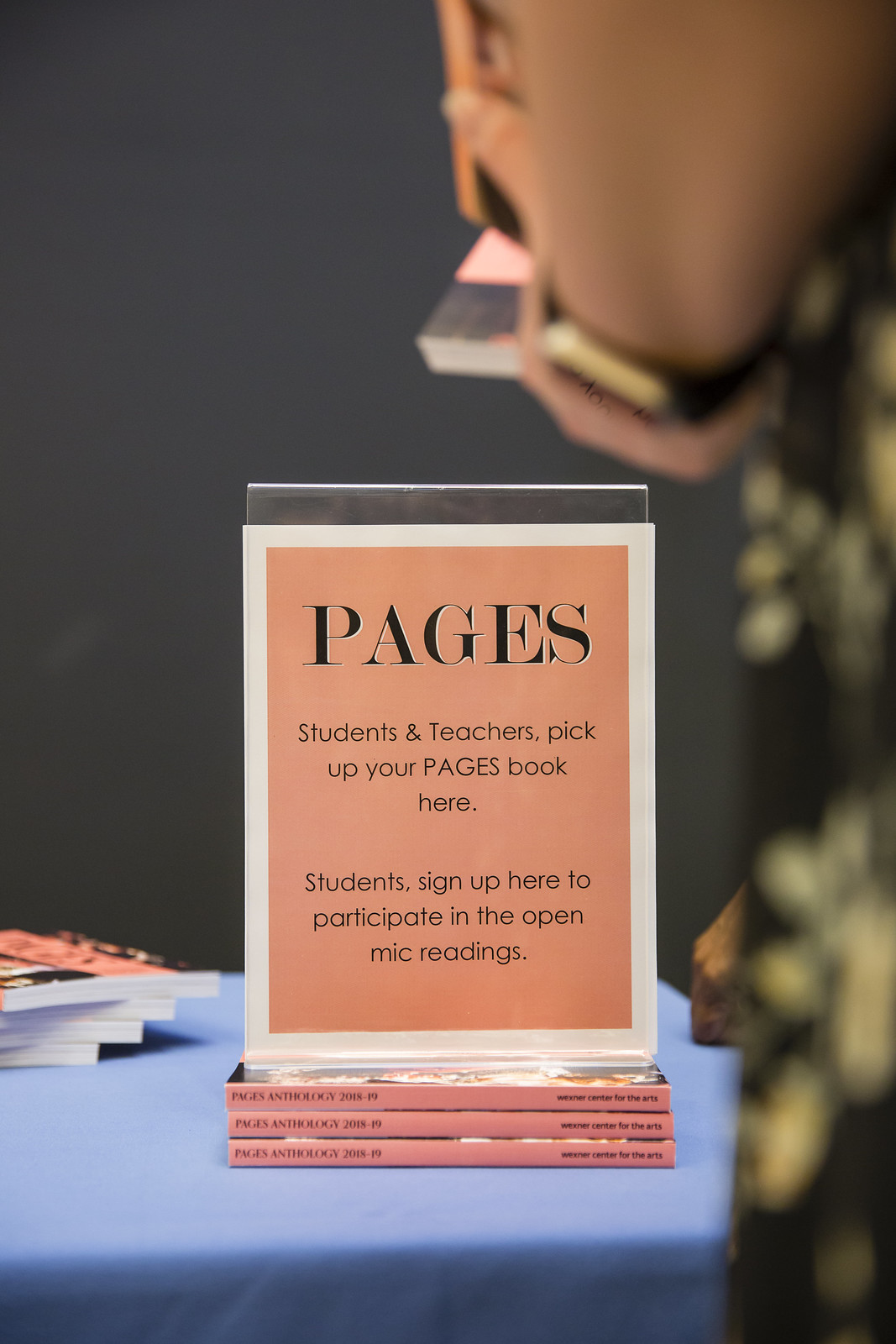This is a photo capturing a book event, featuring a stack of three books titled "Pages Anthology 2018-19" by the Wexner Center for the Arts, placed on a blue tablecloth-covered table. Positioned on top of these books is a sign in a plastic holder that reads: “Pages. Students and Teachers pick up your Pages book here. Students sign up here to participate in the open mic readings.” The left side of the image shows more copies of the same book. The backdrop appears to be a black wall. To the right, there is a slightly blurred outline of a person wearing a watch, holding one or two copies of the book, with another person’s hand resting on the table near the stacked books. The scene suggests that people are gathered, likely picking up their copies of the book and possibly signing up for the open mic readings.